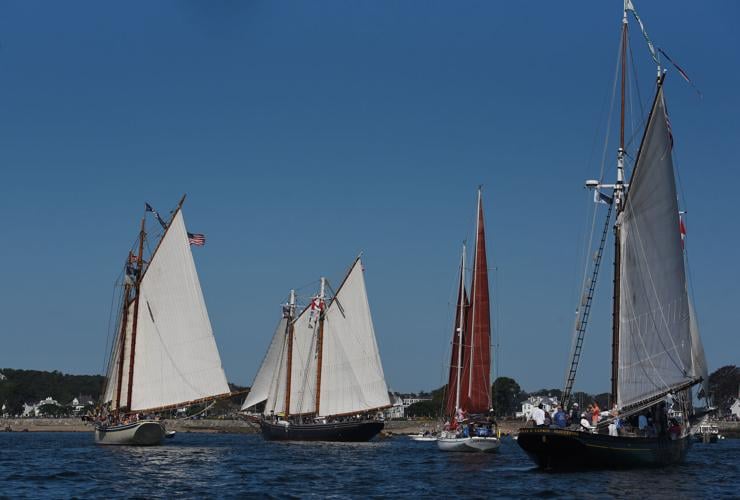In this vibrant daytime photo, against a backdrop of a bright, cloudless blue sky, four prominent sailboats are gracefully sailing on what is likely the ocean, given the calm water with tiny ripples. The background is adorned with a line of trees and a distant shoreline, featuring some buildings visible. 

The sailboats, the main focus of the picture, are detailed with distinct characteristics:
- The first boat on the far left sports white sails and a blend of white and navy on its hull. It features two large wooden masts and an American flag at the top, along with another flag to the left. The boat's base appears gray, and it is bustling with multiple people onboard.
- The second boat, slightly to the right, separated by the dark blue ocean, also has white sails and wooden masts. Its hull is a dark color, possibly black or dark blue, and its sails are fully set.
- The third boat, centrally positioned, stands out with its vibrant burgundy red sails and a white hull, resembling that of a catamaran. This boat too has several people visible on deck.
- The fourth and largest boat, situated on the far right, features gray sails and a black hull. Its two wooden masts are adorned with flags, and it is populated with figures including a man in a blue shirt at the bow, along with others dressed in a variety of colors such as black, white, gray, pink, and blue.

The image captures a serene yet lively maritime scene, filled with the elegance and motion of sailboats under a bright, sunlit sky.